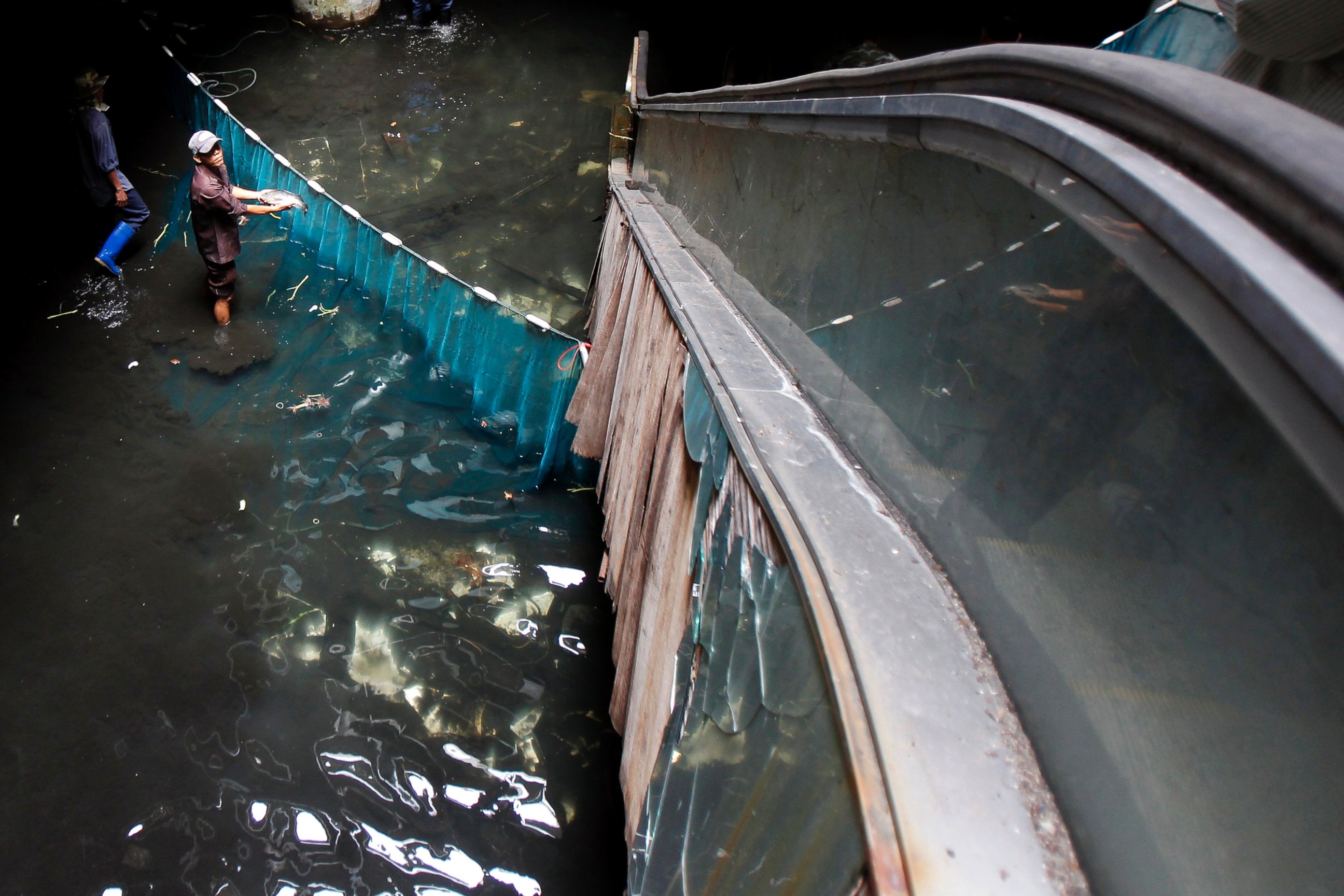The photograph, taken in color and landscape orientation, depicts an indoor scene where we are looking down from the second story of a building at a flooded lower level. In the upper left-hand corner, two men, appearing to be of Asian descent, are standing knee-deep in the muddy, brackish water. One holds an aquatic animal, while a blue curtain, adorned with buoys, stretches across the scene. The right side of the image features a bridge-like structure reminiscent of an escalator, with a visible armrest leading down into the water. The side walls appear aged and deteriorating, with a sheer drop-off revealing a broken surface below. The overall composition conveys a sense of realism and representationalism, highlighting the unexpected indoor flooding and the activities of the men amidst the scene.